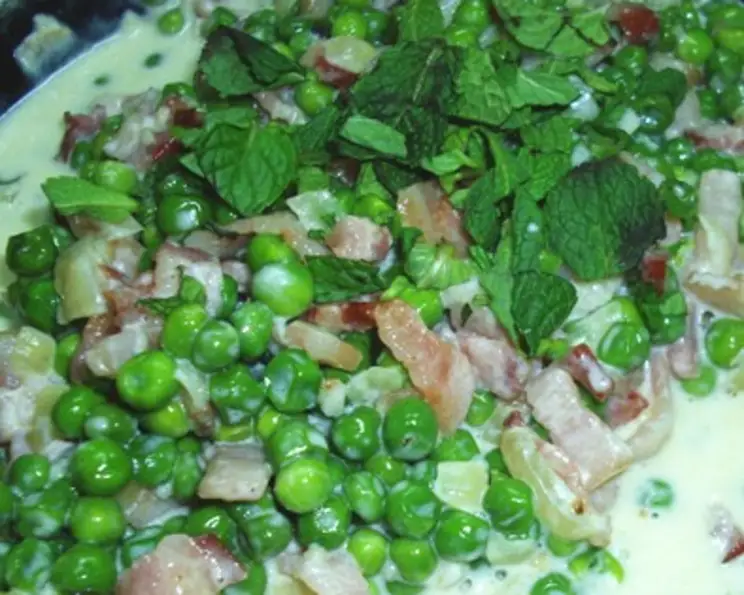This extremely close-up, rectangular image captures a rather blurry and unappealing view of a soup. Dominating the entire frame, the soup's creamy, light green broth envelops an assortment of green peas, which appear slick and moist due to the broth's texture. Scattered throughout the mixture are pieces of bacon or thinly sliced meat, some of which are a lighter brownish-white color, while others are darker red, possibly indicating a different cut or even red onion. Sprinklings of green leaves, which might be arugula or mint, add a touch of vibrant color amidst the creamy concoction. The soup's edges are indistinct, leaving most of the image filled with food chunks and creamy broth, and only a hint of a black background peeks through in the top-left corner, suggesting the edge of a bowl or serving dish. Despite its less-than-appetizing appearance, the blend of ingredients might still hint at a delicious flavor.